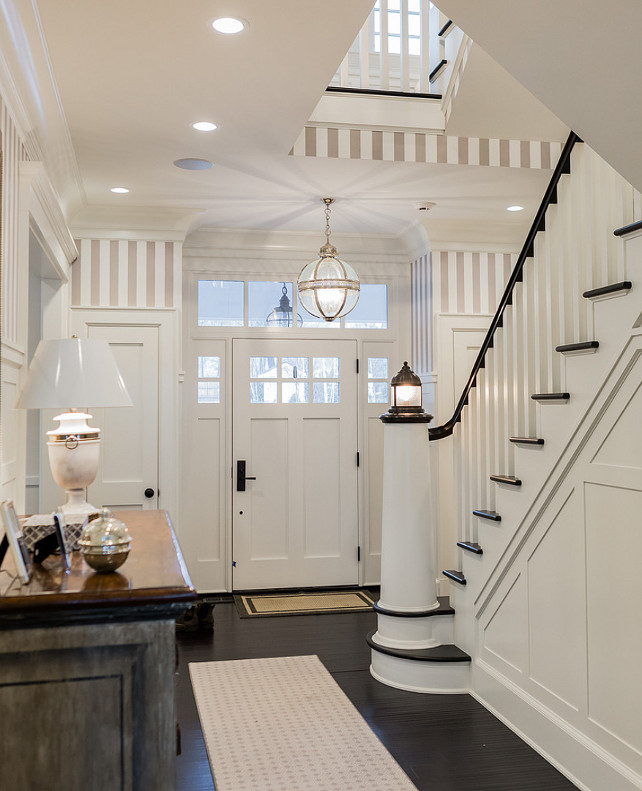The image captures the front foyer of a spacious and modern home, adorned with a distinct nautical theme. The foyer is characterized by its predominantly white palette, contrasted with black accents, creating a crisp and clean aesthetic. Central to the image is the front door, flanked by window lights and crowned by a large, elegant glass chandelier with gold trimming, which sets a welcoming tone.

Upon entering, a dark floor is immediately noticeable, highlighted by a white runner rug that aligns harmoniously with the room’s white decor. The focal point of the foyer is a striking white staircase trimmed in black, resembling a lighthouse with creative touches that enhance the nautical feel. This staircase leads upwards, suggesting the presence of multiple levels within the home.

To the left of the entrance stands a wooden side table adorned with a white lamp and minimalistic decorative items, including a round silver ornament and some framed photographs. Above, inset pot lights in the ceiling provide a glowing illumination throughout the large and inviting space. The foyer's minimal but purposeful decor lends itself to a modern and open atmosphere, emphasizing both the expansive design and the detailed nautical elements.